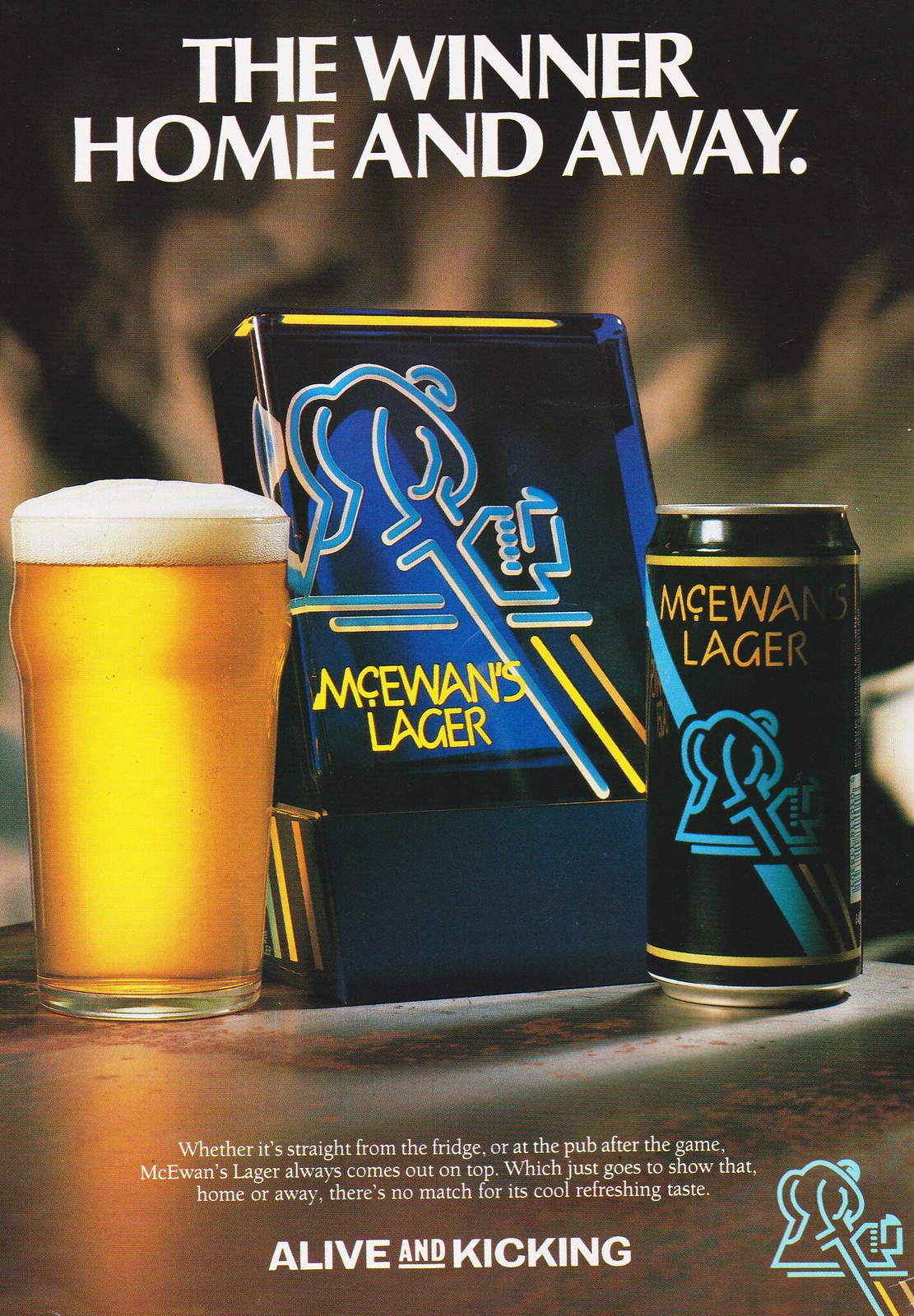The image is a detailed advertisement for McEwen's Lager beer, prominently featuring vibrant colors and several key elements. At the top of the ad, bold white text on a brown background declares, "The Winner Home and Away." Central to the image is a sign with a blue caricature of a hockey player holding a stick. This sign, which reads "McEwen's Lager" in yellow letters on a blue background, is flanked by two beverages: a glass of frothy beer on the left and a can of McEwen's Lager on the right. The can, decked in dark blue or black with yellow lettering and light blue logos, mirrors the central hockey player silhouette. Below the main sign, a tagline in white reads, "Alive and Kicking," and just above it in smaller white print, the text says, "Whether it’s straight from the fridge or at the pub after the game, McEwen’s Lager always comes out on top, which just goes to show that home or away, there's no match for its cool, refreshing taste." The objects are arranged centrally on a multicolored table with shades of gray, white, yellow, orange, blue, black, silver, and tan, emphasizing the advertisement's vibrant and engaging design.